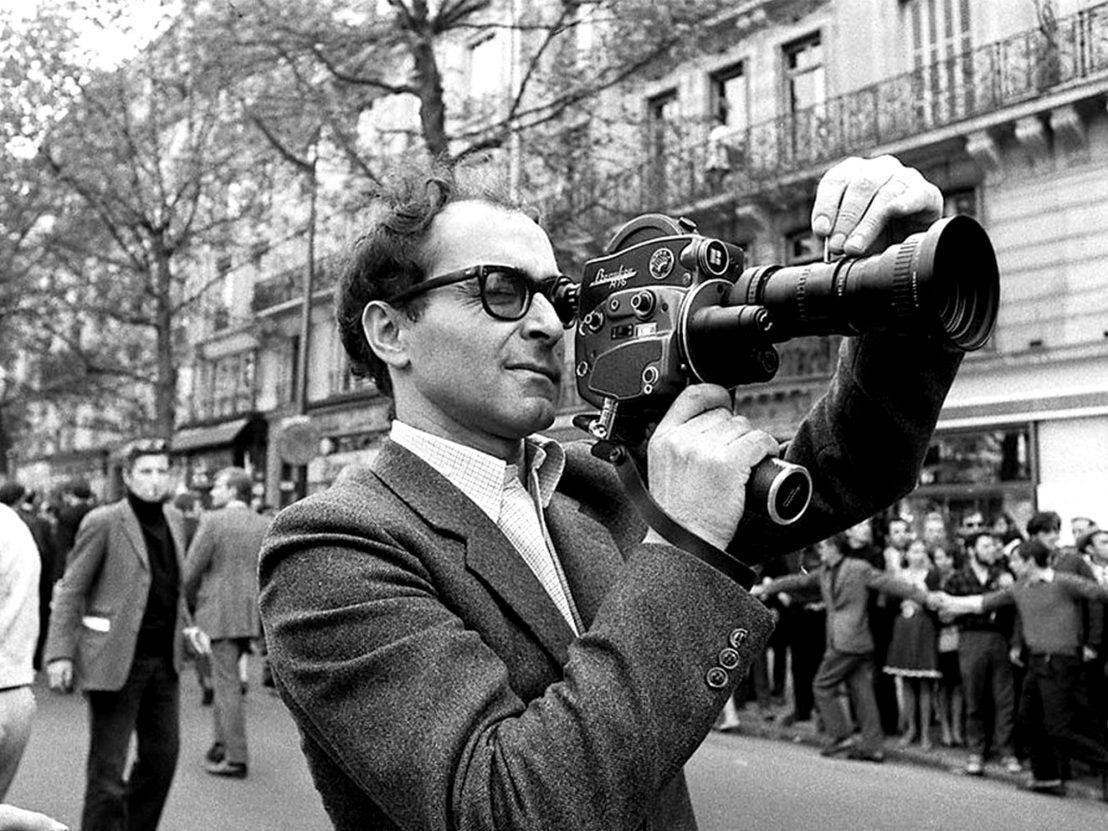In this black-and-white photograph, likely taken in the late 1970s or early 1980s, a man in the foreground is the central figure. He is dressed in a dark blazer and white shirt, his short dark hair and dark-tinted glasses giving him a distinct appearance. He is peering through the viewfinder of an old, handheld video camera, which he holds by a bar beneath the device while his other hand steadies the lens. His intense concentration is evident as the eye behind the glasses appears to be squinting.

The scene unfolds on a bustling city street, lined with apartment buildings that feature railings on the second stories. Trees dot the sidewalk, adding a touch of nature to the urban environment. A dense crowd is gathered on the sidewalk, resembling a large congregation for an event of some significance. The crowd is being held back by several men who interlock their arms to form a human barricade, preventing them from spilling onto the street. Additional men in suits stand off to the side, possibly overseeing the scene or serving some official capacity. The overall atmosphere is one of controlled chaos, with numerous people milling about, all under the watchful lens of the camera operator.